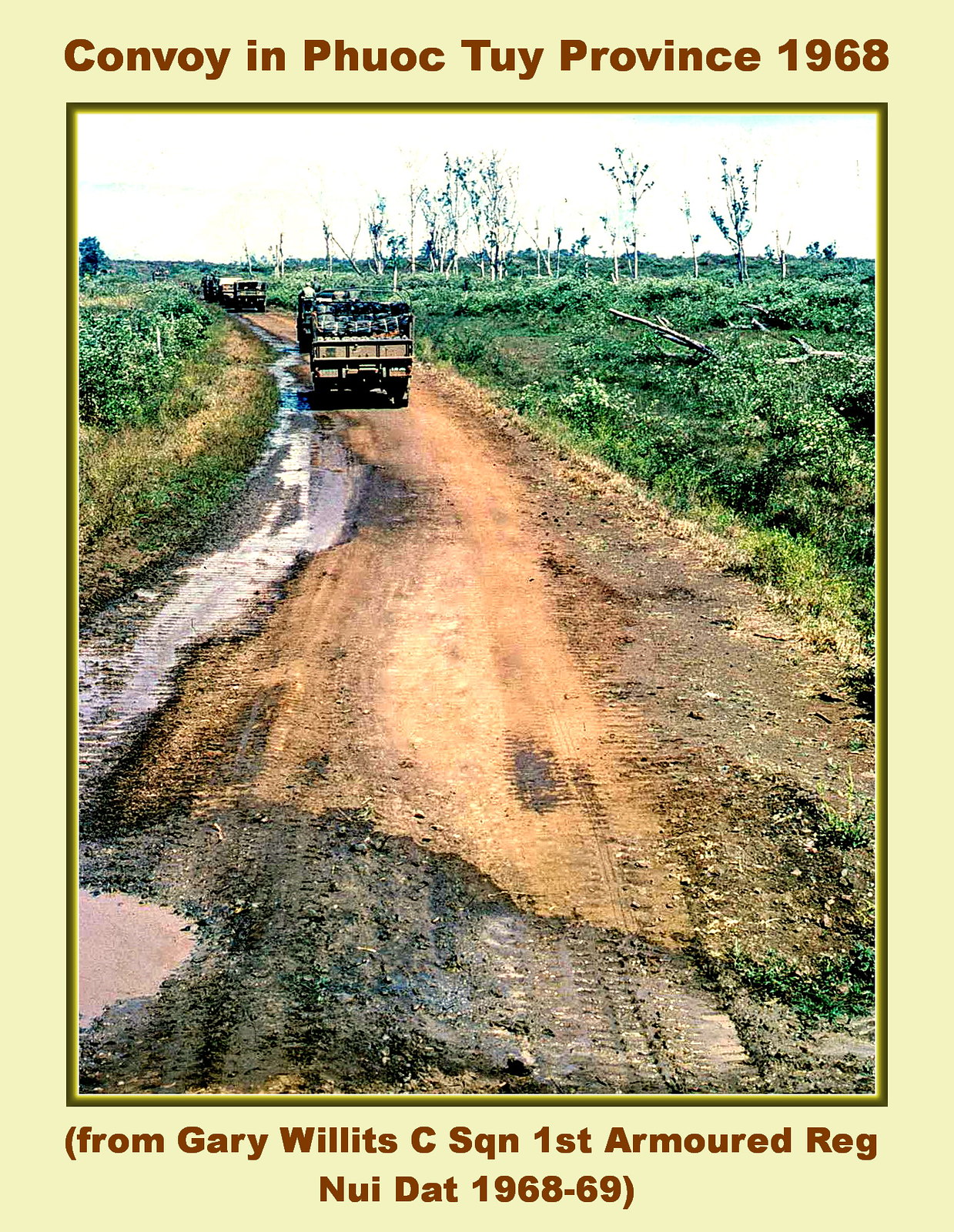The photograph captures a dirt road flanked by lush greenery and sparse, skinny white trees in the distance. The left side of the road is particularly muddy with pools of water. In the middle distance, there are beige armored military vehicles, though they appear somewhat blurry due to the distance. The sky above is extremely bright, almost washed out with no visible details. The top of the image is marked with the text "Convoy in Phuc Thuy Province, 1968," and the bottom reads "From Gary Wiltus, C. Squinn, 1st Armored Reg., Nui Tat, 1968-69."